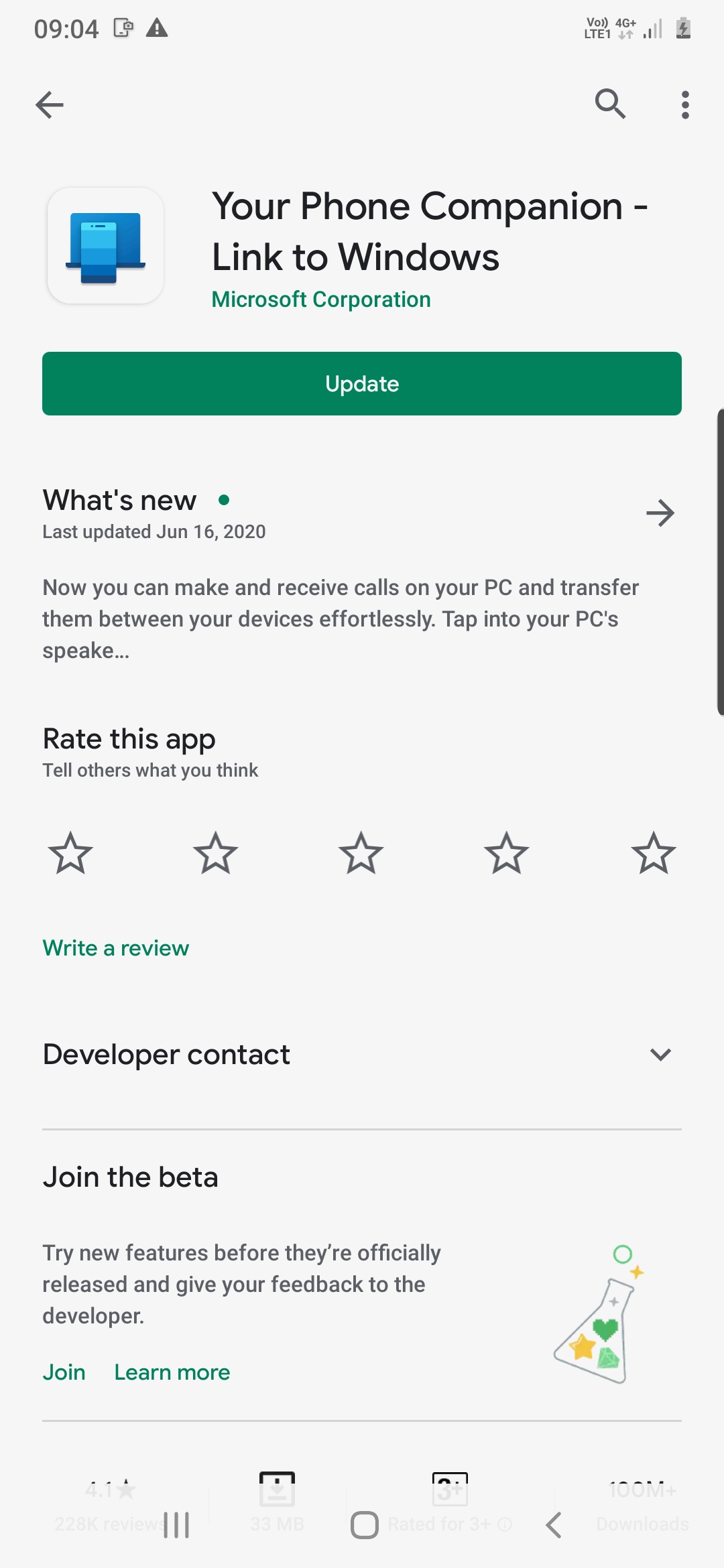**Detailed Caption:**

In this image, we see a screenshot of a web page captured from a tablet device. The top portion displays a status bar showing the time, "09:04," accompanied by various icons symbolizing settings. The status bar indicates a strong phone signal and reveals that the device is using 4G for internet connectivity. Just below this, on the right side of the screen, there's a magnifying glass icon signifying the search function, followed by three vertical dots suggesting access to additional options or menus.

Beneath this, a blue icon is visible, accompanied by the text "Your Phone Companion - Link to Windows" in black letters against a light gray background. This section is identified as a product of Microsoft Corporation. Directly below, a prominent green "Update" button is displayed. The "What's New" section provides the latest update date as June 16, 2020, and describes new features: the ability to make and receive calls on a PC and transfer them seamlessly between devices, with partial text trailing off with an ellipsis.

Following this, a section prompts users to "Rate this app," featuring a five-star rating system with no stars currently selected, and an invitation to "Write a review" via a clickable button. Further down, the text "Developer contact" is highlighted in bold black letters, along with a dropdown menu that remains collapsed.

The next segment invites users to "Join the beta," emphasizing in gray letters the opportunity to try new features before their official release and provide feedback to the developers. Two buttons follow - "Join" in aqua-colored letters and "Learn more" in the same color scheme.

At the bottom right of the screen, there's a distinctive icon resembling an Erlenmeyer flask adorned with a green heart, a yellow star, and a light green heart.